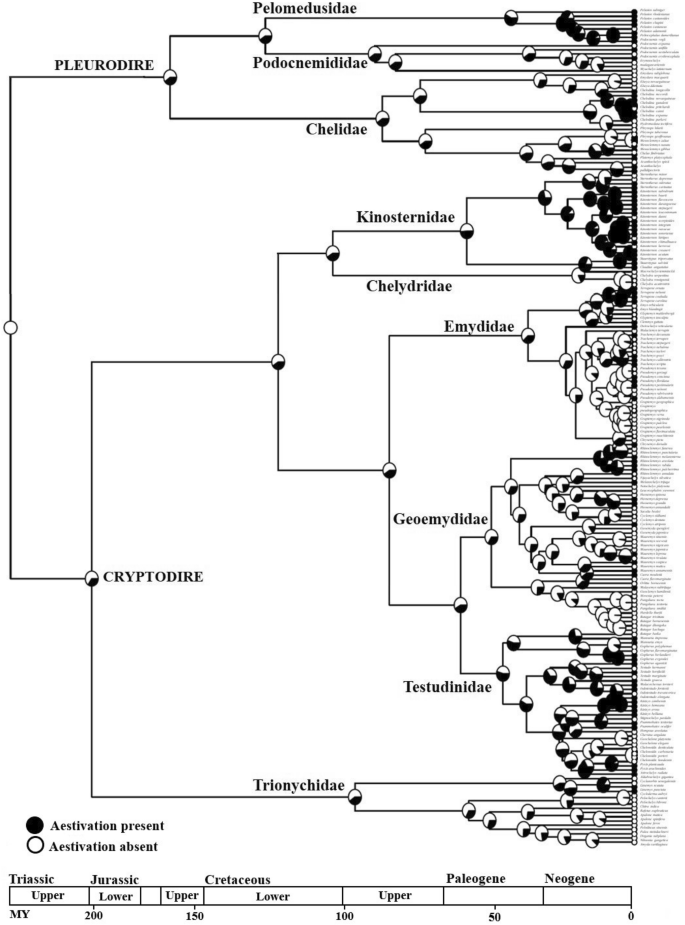This intricately detailed black-and-white infographic, set against a white background and oriented vertically, is a complex flowchart that visually outlines scientific classifications, possibly related to turtle taxonomy. On the left side, the diagram begins with two main branches labeled "Plurodire" at the top and "Cryptodire" at the bottom. From these points, an extensive series of branching lines emerge, resembling a family tree or tournament bracket.

Under "Plurodire," the diagram splits into subcategories such as "Palomedusidae," "Podosimedidae," and "Chelidae," where each branch leads to smaller circles and further subdivisions. Similarly, "Cryptodire" breaks down into sections like "Chenosternidae," "Chelidrae," "Amydidae," "Geomydidae," "Testudididae," and further onto "Triona Chelidae."

On the right side, there are numerous horizontal lines interspersed with small, labeled black and white circles. These circles refer to a key at the bottom left indicating whether "estivation" is present (black) or absent (white). Below this, a chronological bar chart lists geological periods such as Triassic, Jurassic, Cretaceous, Paleogene, and Neogene, marked by labels like "upper" and "lower" and numerical values (e.g., MY 200, 150, 150, and 0). The diagram's far-right side features exceedingly tiny, mostly illegible text alongside vertical lines that extend various lengths, indicating different levels of classification or evolutionary timelines.

Overall, the infographic is a detailed line-art representation that uses numerous scientific terms, challenging the reader's comprehension but vividly portraying the complexity of the depicted data.